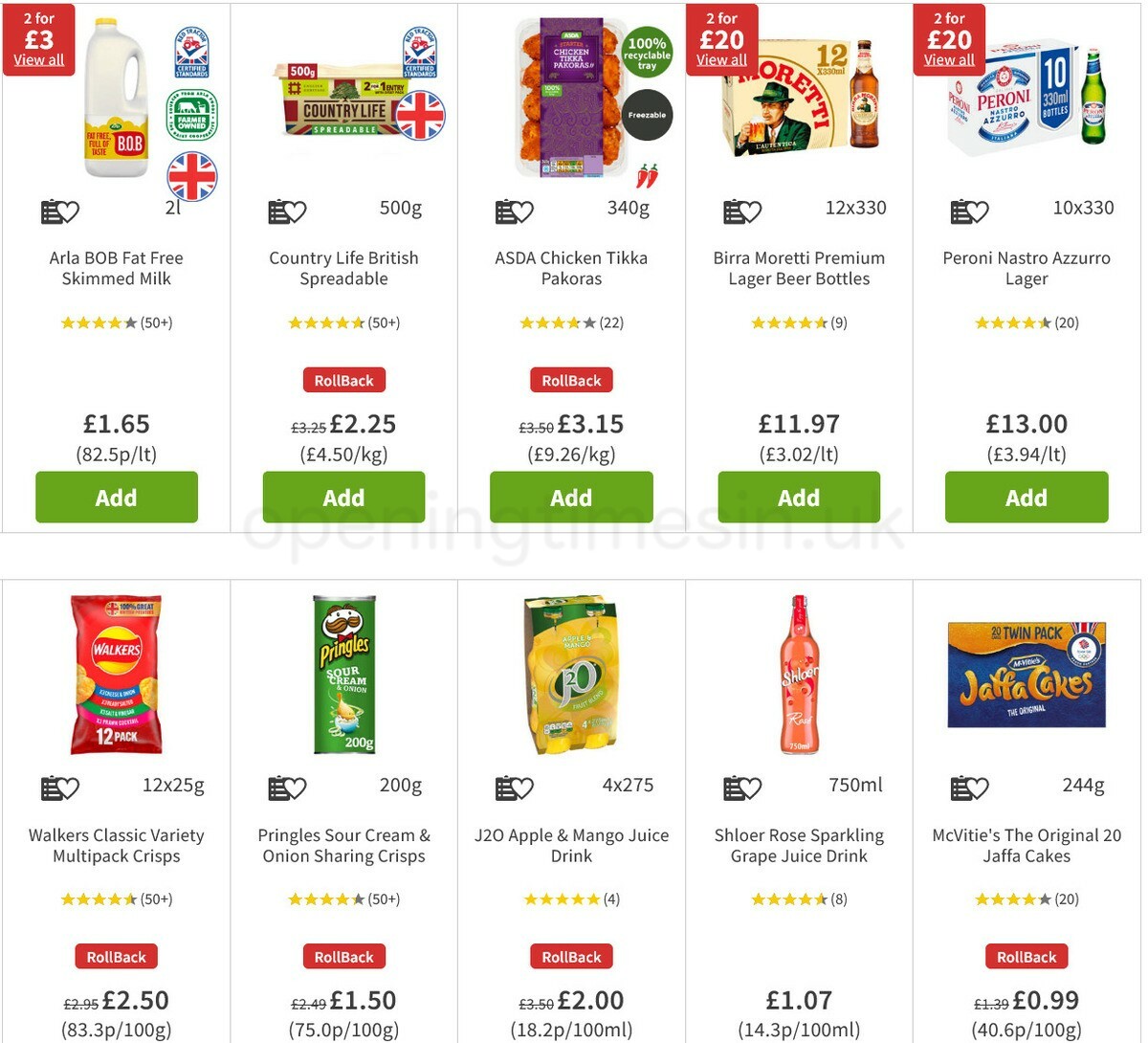The image appears to be a screenshot from an online grocery store website, displaying a grid of products available for purchase. There are ten vertical rectangles arranged in two rows of five. Each rectangle features a different food item along with detailed information and an "Add" button for easy selection.

**Top Row:**
1. **Milk**: This is a jug of Arla Bob fat-free skim milk with a yellow label at the bottom that says "Bob." It features symbols on the right side, including a circle with a British flag and a green icon with a cow indicating it is farmer-owned. The product has a rating of four out of five stars and is priced at £1.65. At the bottom, there's a green "Add" button in white text.

**Other Recognizable Products:**
- **Butter or Margarine**
- **Beer**
- **Grape Juice** (possibly sparkling grape juice)
- **Pringles** (Sour Cream and Onion flavor)

**Additional Details:**
Each product listing includes a price, an average rating out of five stars, and an "Add" button in a green rectangle with white text, enabling users to quickly add items to their cart. The products are diverse, including dairy, snacks, beverages, and more, accommodating various shopping needs.